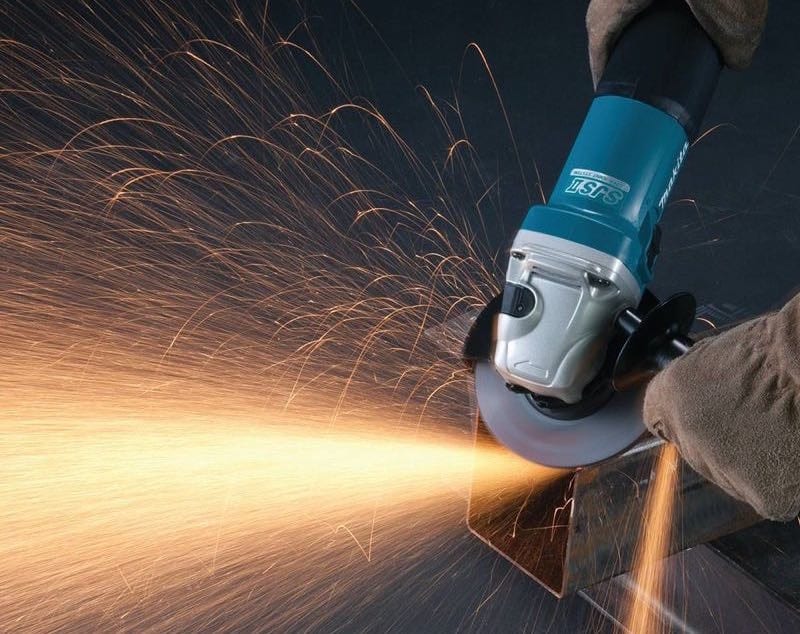In this vivid photographic image, a person wearing brown gloves is seen operating an electric saw. The saw's design includes a light blue cylindrical body marked with the letters "SRS" and a gray tapered front section meeting the gray saw blade. The scene is dynamic, with a multitude of bright, triangularly-shaped sparks erupting from the point where the blade contacts a metal surface. The process could be occurring either indoors or outdoors, as the focus is tightly on the intense interaction between the saw and the metal. The operator's hands are firmly holding the saw, suggesting precision and control as they either cut through or sharpen the metal, emphasizing the vigorous and meticulous nature of this task.